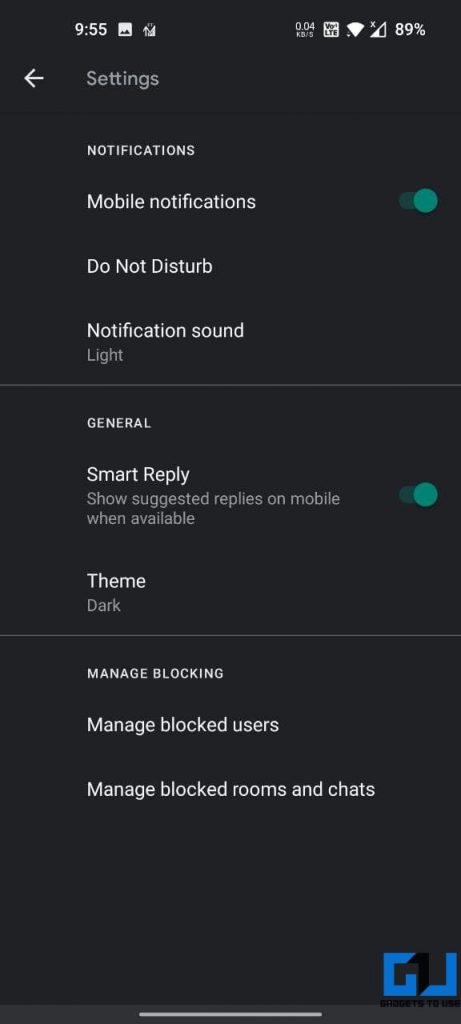A detailed screenshot taken from a mobile device shows the user navigating through their phone's settings interface, which is not formatted like an iPhone. At the top left of the screen, the time is displayed as 9:55 AM, alongside an indistinct image logo and another unrecognizable app notification icon. On the top right, the status bar displays a data transfer rate of 0.04 kbps, an LTE symbol, a Wi-Fi icon, a mobile data strength indicator with a small 'X' above it suggesting no data connection, and a battery percentage of 89% without an accompanying battery icon.

In the main settings interface, "Settings" is prominently displayed at the top, with a left-pointing arrow for navigating back. Directly below, the "Notifications" section is visible, indicating that mobile notifications are toggled on. Other settings include "Do Not Disturb," and "Notification Sound" set to "Light." The "General" section follows, featuring options such as "Smart Relay," which is toggled on, and "Show suggested replies on mobile when available," also toggled on. The interface is set to a dark theme. Further down, there are options for managing blocked users, rooms, and chats.

In the bottom right corner, there is a watermark with a symbol incorporating the letters 'G' and 'U', and the text "Gadgets to Use." The overall interface is characterized by a gray background with green accents.